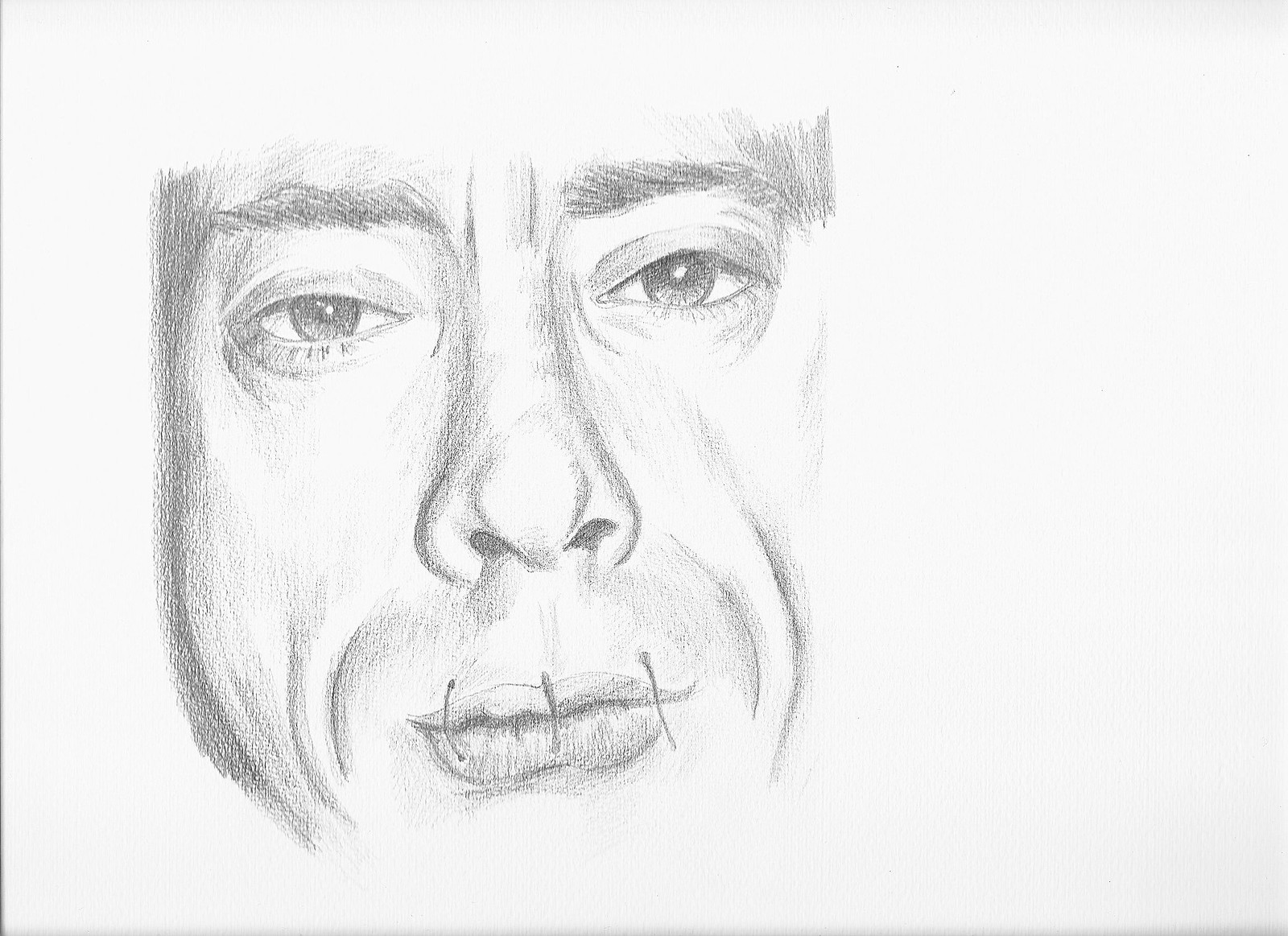This detailed pencil sketch, drawn on a horizontal piece of white sketch paper, depicts the face of an older man with a neutral yet somber expression. His thick, bushy eyebrows sit above sad and perfectly rendered eyes that reflect light, giving them a lifelike quality. His face, shaded on the left side and along the edges, conveys depth and rugged texture, with pronounced lines around his mouth and cheeks. The man's long, wide nose leads down to his lips, which are sewn shut with three stitches - one at each corner and one in the middle, possibly symbolizing themes of censorship. The drawing abruptly ends at his chin and the top of his forehead, leaving a powerful, haunting impression.